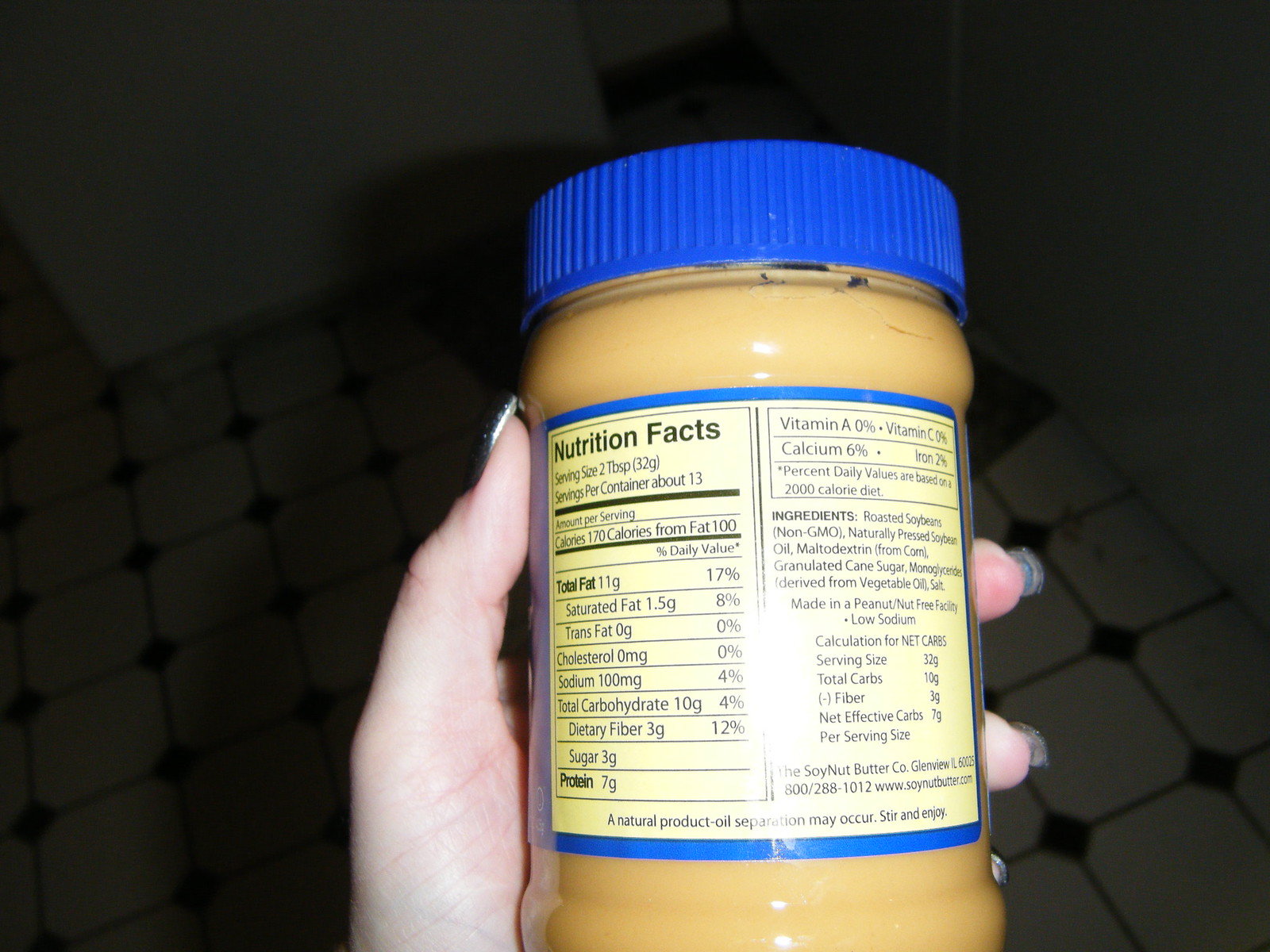In this photograph, a white female is holding a clear jar of peanut butter in her left hand, adorned with long nails painted in glittery polish. The jar features a dark blue, screw-on circular lid and a prominently displayed square sticker with nutritional facts, bordered by blue and filled with yellow detailing. The nutritional label indicates a serving size of 2 tablespoons (32 grams), with approximately 13 servings per container. The peanut butter supplies 170 calories per serving, with 100 calories from fat. It contains 11 grams of total fat (17%), including 1.5 grams of saturated fat (8%), 0 mg of cholesterol, 100 mg of sodium (4%), 10 grams of total carbohydrates (4%), 3 grams of dietary fiber (12%), 3 grams of sugar, and 7 grams of protein. The vitamin content includes 0% vitamin A, 0% vitamin C, 6% calcium, and 2% iron.

The background of the image is dimly lit, suggesting the room lights are off, with the peanut butter jar illuminated by the camera's flash. The floor features white tiles with black diamond shapes at the corners of each tile, adding a striking geometric pattern to the scene. The woman's thumb and the tips of her fingers are visible, encircling the jar firmly.